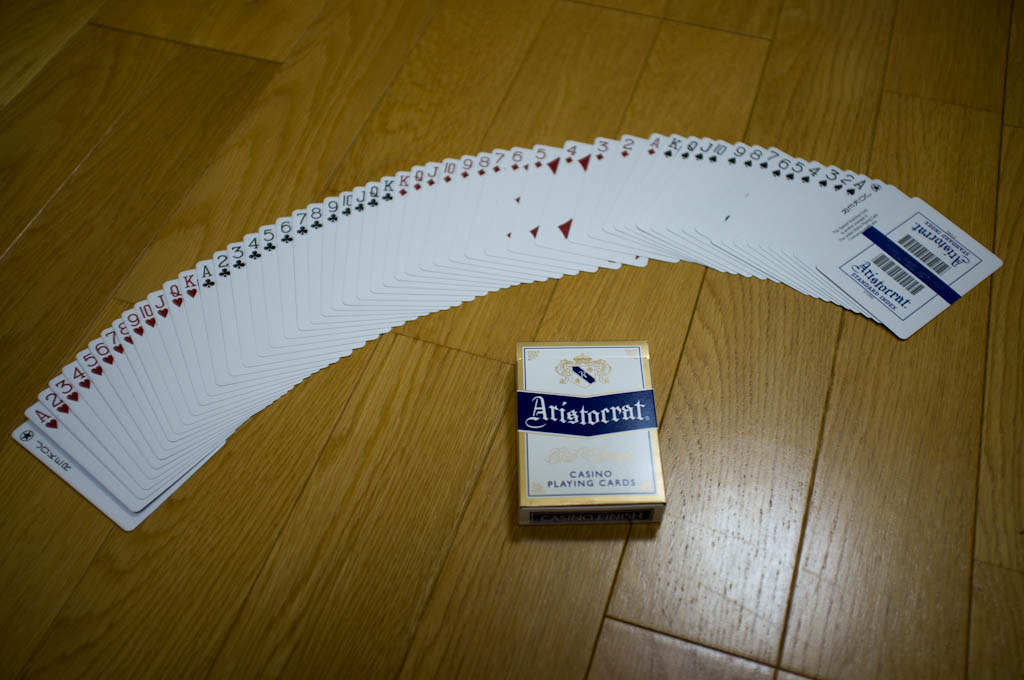This photograph showcases a deck of playing cards meticulously spread out in an elegant arch formation, with each card overlapping slightly to form a single row. The arrangement allows only the upper edges of the cards to be visible, displaying the card's number or symbol and suit. For example, the ace card reveals its 'A' and heart symbol. In front of this arched display, the deck's box is prominently placed, featuring the brand name "Aristocrat" in a classic Old English font, along with the words "casino playing cards" within a white rectangle bordered in gold. The cards are sorted by suit, presenting hearts, clubs, diamonds, and spades in a precise order.